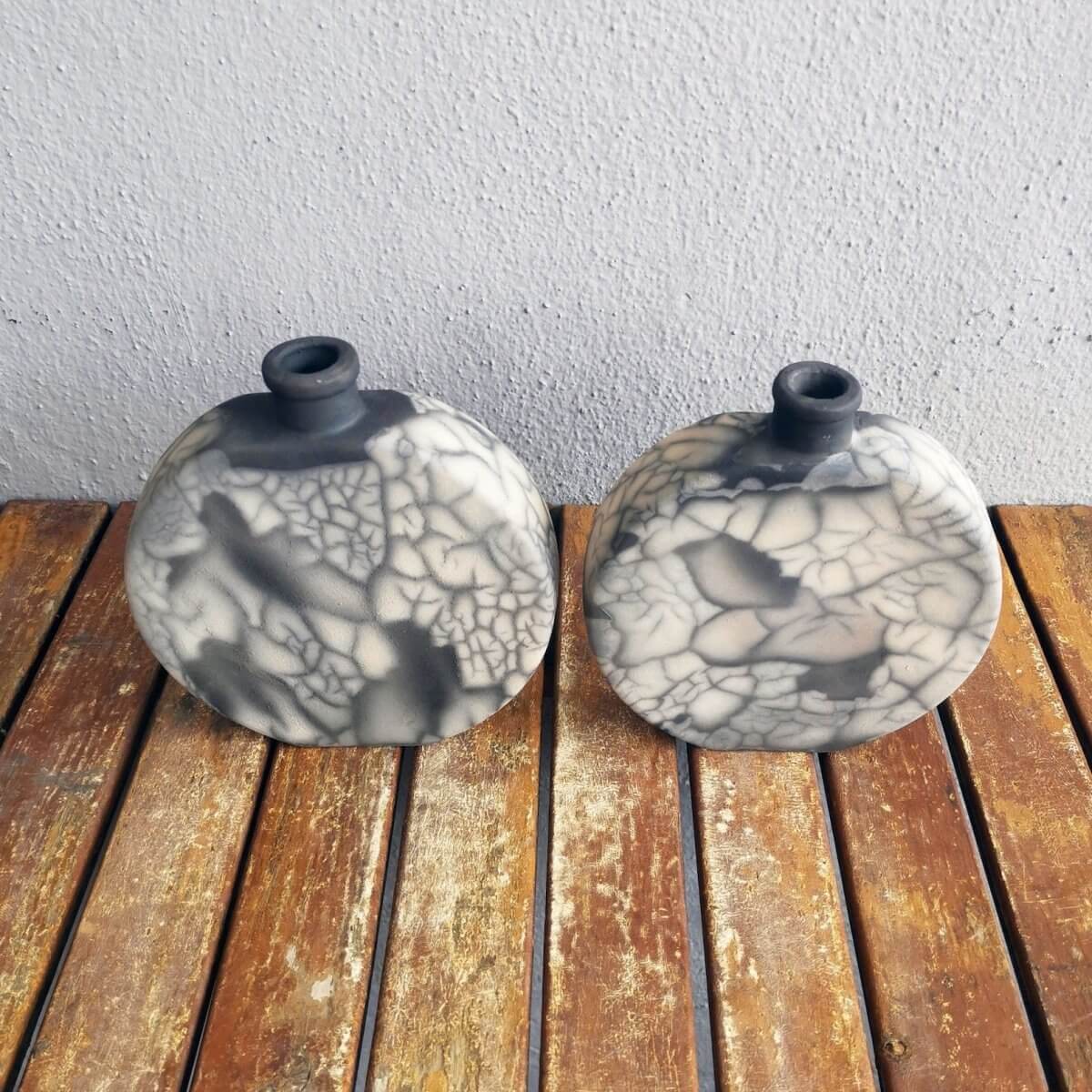The image captures a pair of identical vases placed side by side on weathered brown wooden slats with visible gaps between them. The vases are predominantly white with gray, marbled patterns that resemble cracks and leaf-like shapes. They are cylindrical in nature, with a circular hollow at the top designed for holding flowers. While they appear round, they are mostly flat on the front and back and rounded on the sides and bottom. The vases are thick, giving the impression they are crafted from a clay-like material. Behind them stands a white, textured plaster wall, adding a rustic background to the photograph.